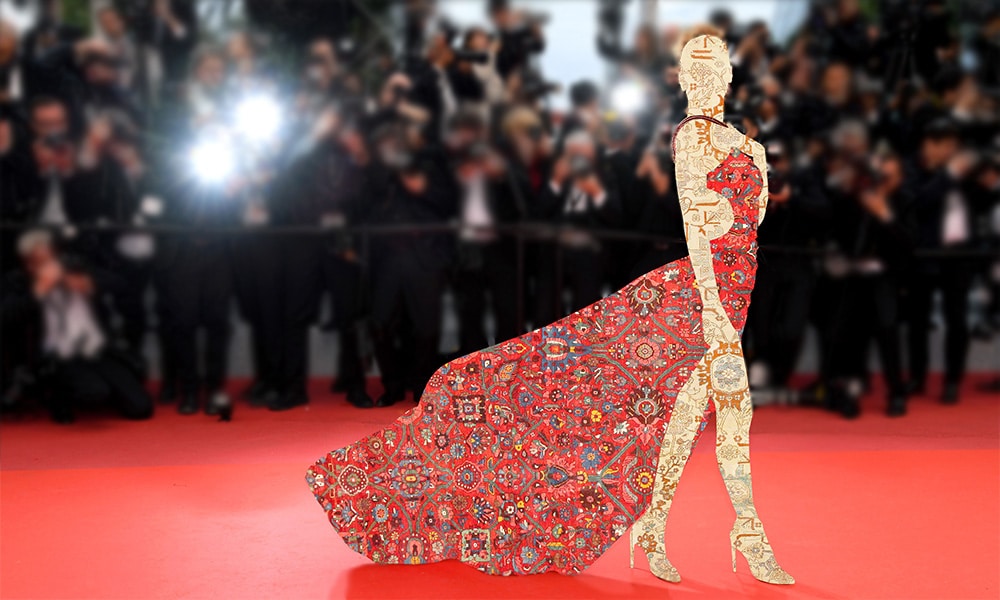In the image, a bustling red carpet event is captured, teeming with paparazzi in the background. Clad in suits, the photographers eagerly snap away, their camera flashes illuminating the scene. However, the focus is on a striking digital creation rather than a real person. The woman depicted wears a stunning, long, flowing red halter dress adorned with various shapes in hues of yellow, blue, and gray. She has light skin and a bald head, with intricate images in brown, beige, and blue adorning her entire body. Completing her look, she stands poised in high heels. The digital artwork seamlessly blends into the vibrant, glamorous atmosphere of the event.